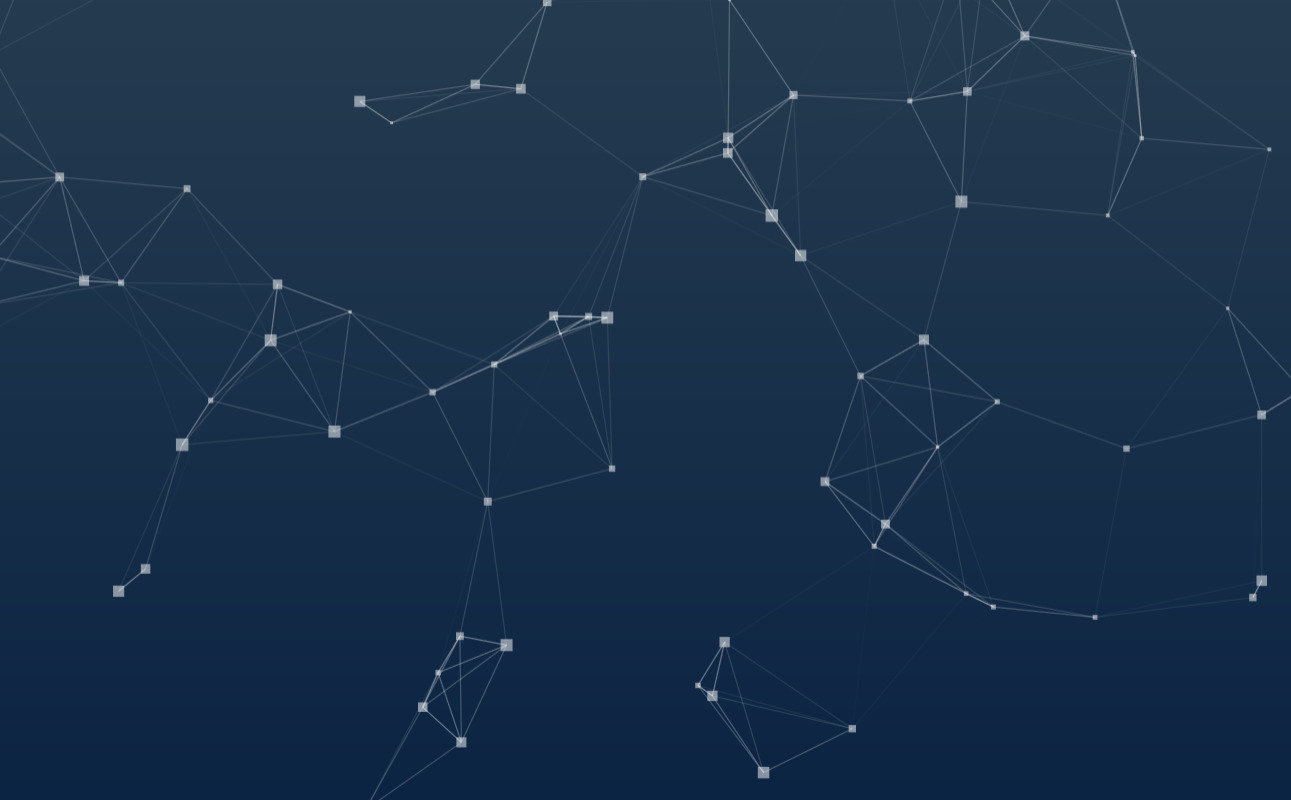The image features an artistic rendition resembling a constellation, set against a dark blue gradient background that lightens toward the top. The composition includes multiple white squares, each interconnected with thin, white transparent lines, giving the impression of celestial formations in a 3D space. The arrangement of these squares and lines does not form a recognizable pattern or specific constellation, but rather an abstract network that evokes the feel of astronomical or astrological maps, reminiscent of elements like Orion's Belt or the Big Dipper. The design highlights the spatial relationships between points, suggesting an intricate, stylized depiction of the night sky.